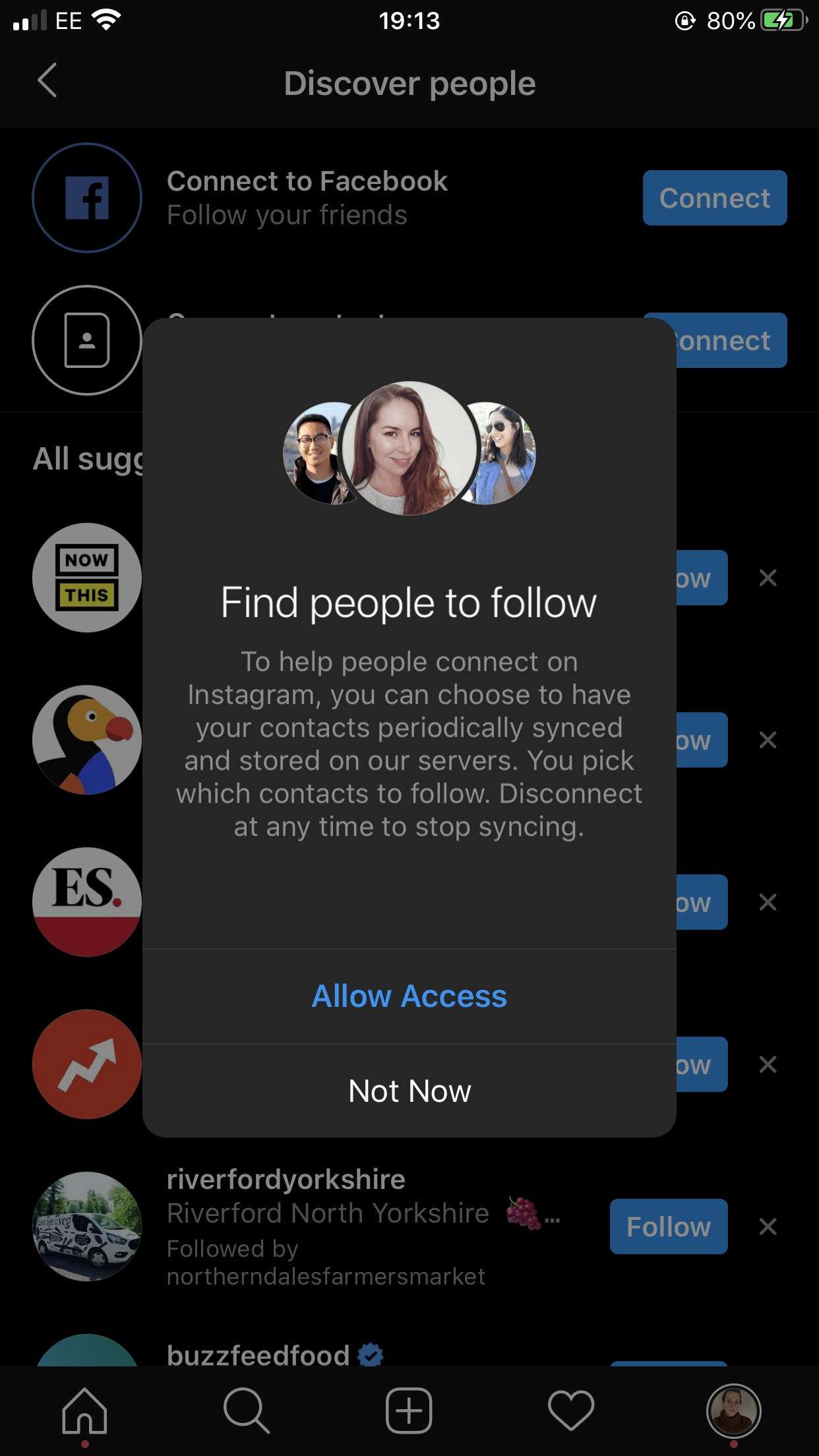A detailed caption for the screenshot could be:

"A screenshot displaying an Instagram prompt, likely triggered upon opening the app. The main focus is on two overlaying rectangular boxes in landscape orientation. The top, active box prompts the user to 'Find people to follow,' offering to sync and store contacts to help users connect on Instagram. This box features two buttons at the bottom: 'Allow Access' and 'Not Now.' Behind this prompt is a secondary box with a black background labeled 'Discover People,' which contains several app icons on the left side. One icon, resembling a duck, is unidentified but appears similar to the 'Dodo' app. Another icon features a stock market symbol. The screenshot appears to have been captured upon initiating or using the app, depicting user navigation and options for enhancing their social network connections."